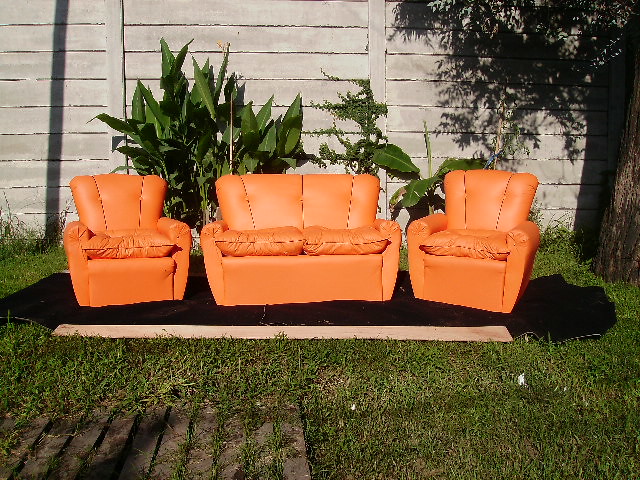In this outdoor photograph, vibrant orange upholstered furniture, consisting of two plush chairs flanking a cozy loveseat, is arranged neatly on a black outdoor rug. These leather-like pieces, in excellent condition, rest on a well-tended patch of short grass with a brick walkway to one side. A sturdy wooden fence with horizontal slats serves as a backdrop, adorned by climbing plants and a sizable potted greenery. A large tree stands to the right, casting intricate shadows that dance on the fence. The scene suggests a tranquil, rain-free backyard setting on a bright, sunny day.